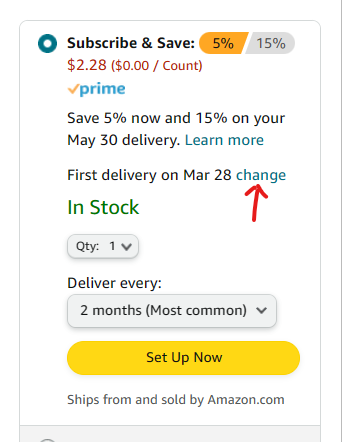A detailed and clean caption for the given image could be:

---
This screenshot displays an Amazon Prime subscription offer. In the top left corner, there's a blue circle with a white dot inside, captioned "Subscribe & Save." To the right, there's "5% / 15%" highlighted in orange, indicating the discount options. Below, the price is listed as "$2.28," and it clarifies "$0.00 / count." An orange checkmark is next to the word "Prime" in blue, emphasizing it's an Amazon Prime product.

Additional text on the page explains: "Save 5% now, 15% on your May 30th delivery. Learn more. First delivery on March 28th." A red arrow is drawn, pointing towards the "Change" option.

Further down, it states in green "In Stock," with "Quantity: 1" following. There is an option to "Deliver every 2 months (Most Common)," followed by a "Set up now" button on a yellow background. The page notes that the item "Ships from and sold by Amazon.com."